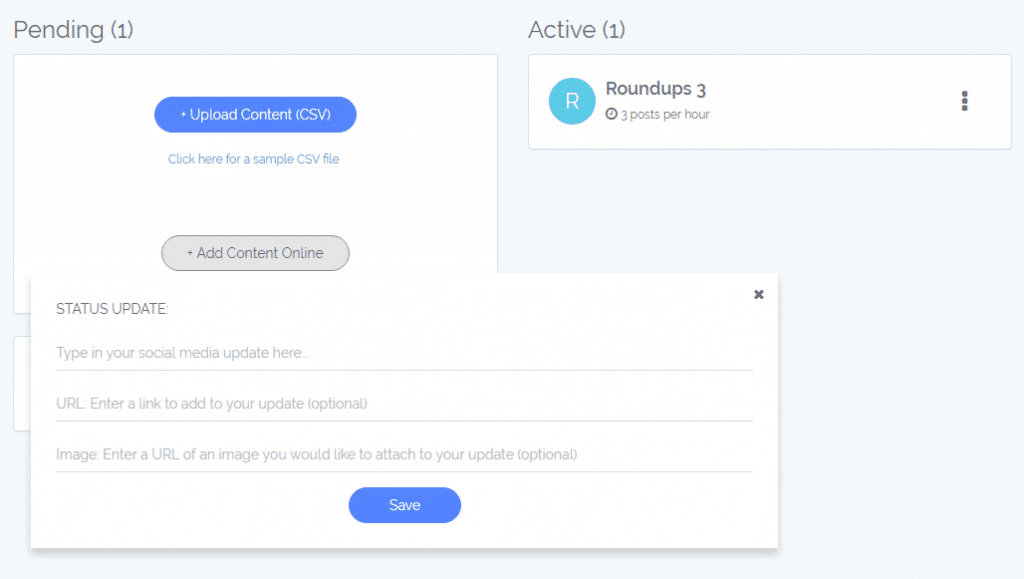Here's a cleaned-up and detailed caption for the image described:

---

The image is a cropped screenshot of an application screen featuring a light blue background. In the top left corner, the text "Pending 1" is displayed in gray. Below this, a white box contains a prominent button labeled "Upload Content CSV," followed by a smaller line of text in light blue that reads "Click here for a sample CSV file." At the bottom of this white box, there is a grayed-out button labeled "Add Content Online."

Moving to the top right corner, the screen displays the text "Active" with a number "1" in parentheses directly below it. Next to this, there is a round profile picture with an "R" on it, which is followed by the text "Roundups 3" and the additional detail "three posts per hour." To the far right, a vertical ellipsis icon (three vertical dots) is present.

In the bottom left corner of the screen, there is a white pop-up window. This window is titled "Status Update" and features the following fields: "Social Media," "URL" with the instruction "enter a link to add to your update" (marked as optional), and "Image," which asks for a URL of an image to be attached to the update (also marked optional). Centered at the bottom of the pop-up is a blue button labeled "Save." Additionally, there is an "X" at the top right corner of the pop-up for closing it.

---